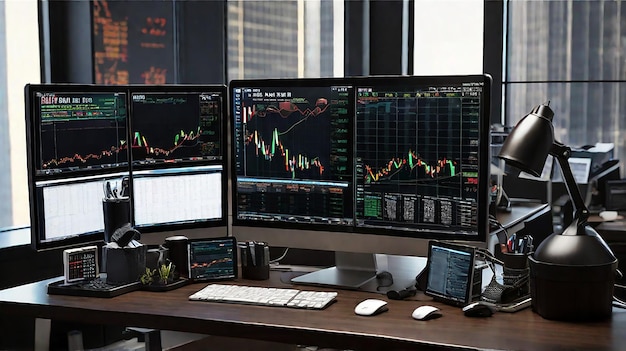The image depicts a detailed office setup with a wooden desk featuring multiple computer screens displaying a variety of multicolored line graphs with red, green, and yellow lines. The monitors are arranged with one vertical screen on the far left and a horizontal screen directly in front of a sleek, white keyboard. This keyboard is accompanied by two mice of different sizes positioned on the right. To the left of the keyboard sits a tray holding a calendar and some planters. On the far left side of the desk rests a digital clock and a cup with pencils, while on the far right, another cup with pens and a small, brushed aluminum desk lamp are placed. The backdrop includes large windows showcasing the city's skyscrapers, though they appear somewhat obscured and the sky is overcast. Additionally, on a side wall in the background, there is an electronic board with orange and red writing, possibly displaying stock prices, though the text is too blurred to be legible. Overall, the image conveys a busy and well-equipped workstation, likely used for stock market analysis.